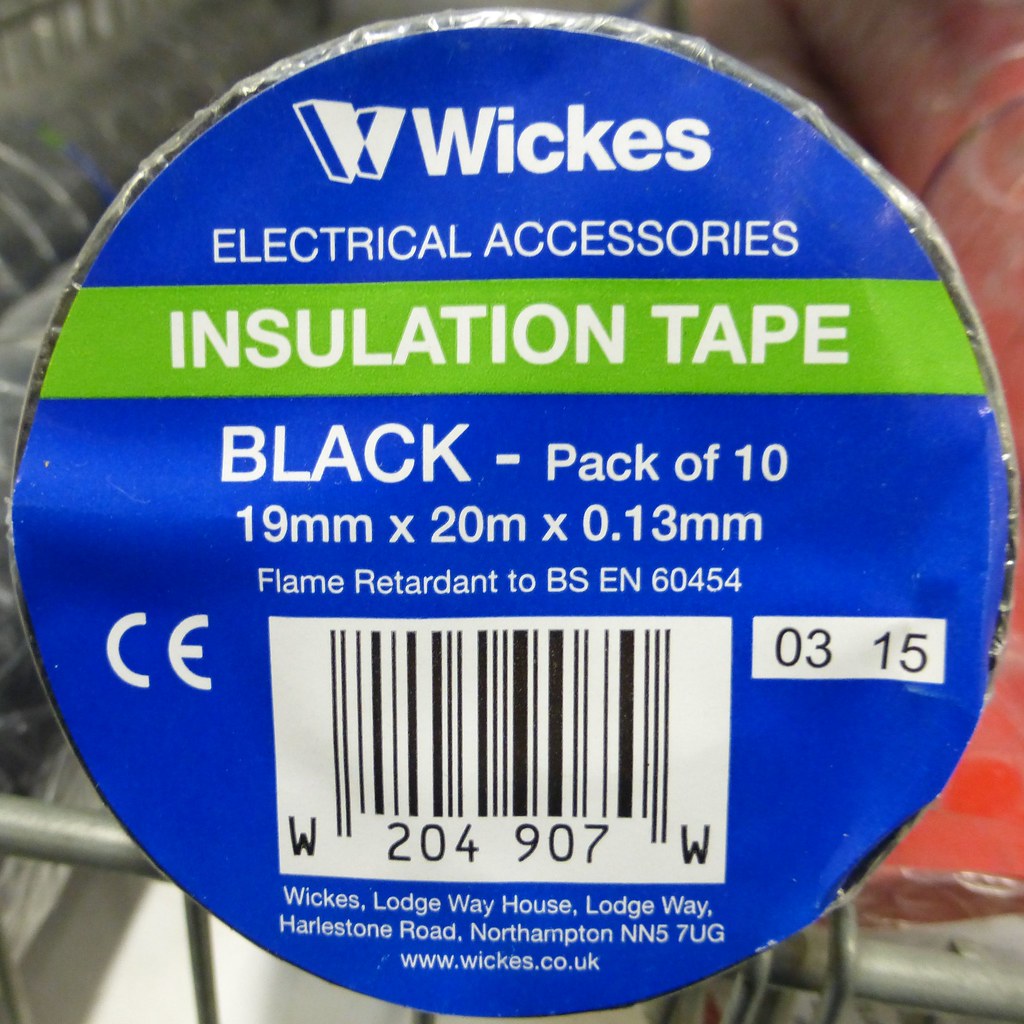The image, square in shape and taken indoors likely in a store, features a close-up photograph of a product positioned in front of the top part of a shopping cart. The product is a package of Wix electrical insulation tape, predominantly housed in a bright blue background with a green band across the middle. In white letters, the top of the packaging prominently displays the brand name "Wix" followed by "Electrical Accessories." The green band contains the text "Insulation Tape," while below, on the blue background, it specifies, "Black Pack of 10, 19mm by 20mm by 0.13mm." The tape is further described as flame retardant, adhering to B-S-E-N 60454 standards. The packaging also includes a barcode, with the CE label to its left and the number 0315 to its right. Below the barcode, manufacturer details read: "Wix, Lodgeway House, Lodgeway Harleston Road, Northampton, NN57UG." This detailed close-up suggests the photograph may be intended to confirm the correct product selection.